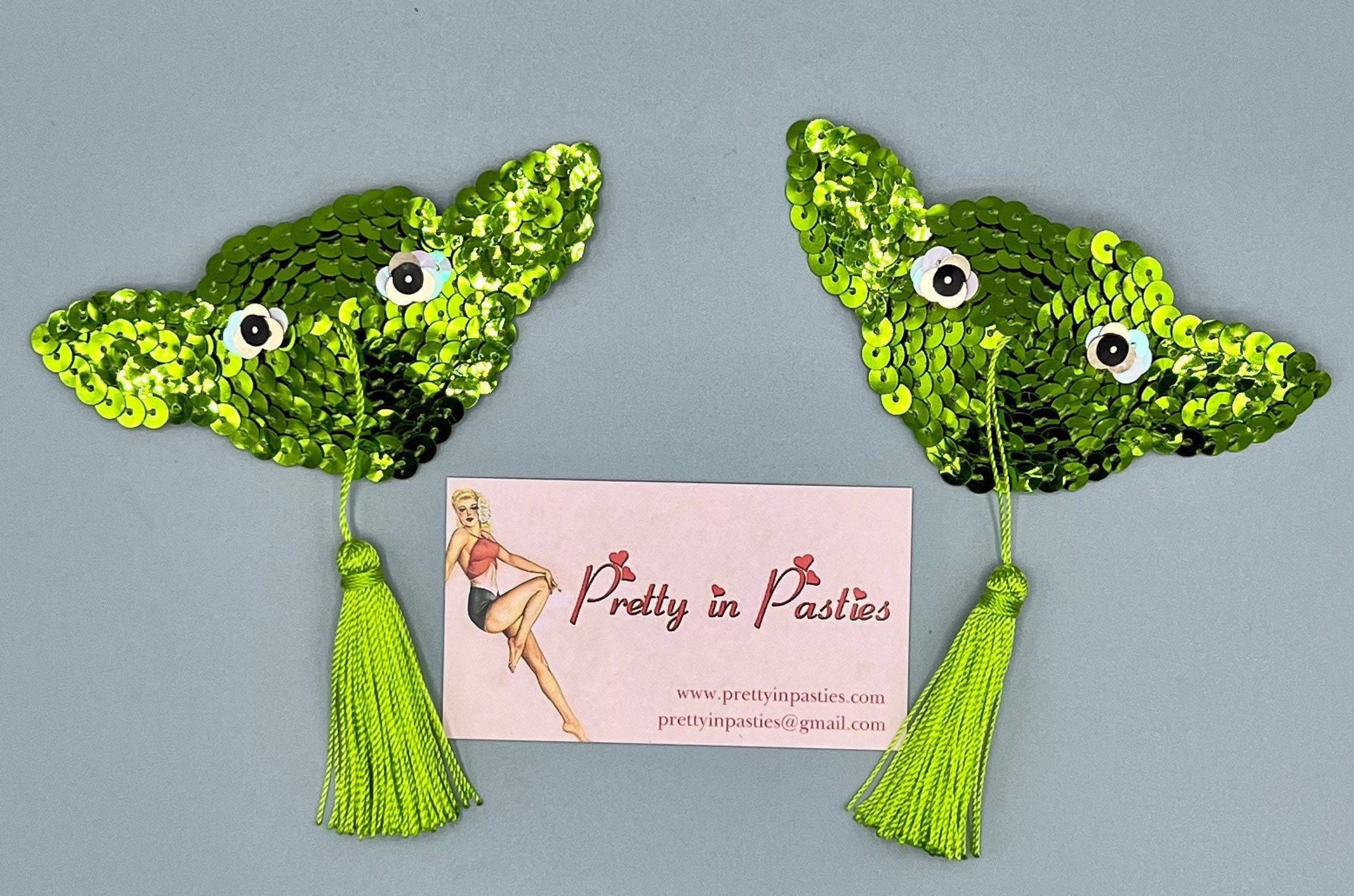In the image, there is a pair of neon green sequined pasties, shaped like Baby Yoda heads, complete with white sequin eyes and black sequin pupils. Each pasty features a green tassel attached by a small string from where Baby Yoda's nose would be. Accompanying the pasties is a pink business card with the text "Pretty in Pasties" adorned with hearts dotting the ‘i’s and ‘P’s. The card also includes contact details: "www.prettyinpasties.com" and "prettyinpasties@gmail.com." On the left side of the card, there's an illustration of a scantily dressed woman in a short skirt and tank top, striking a classic pinup pose with her knee raised.